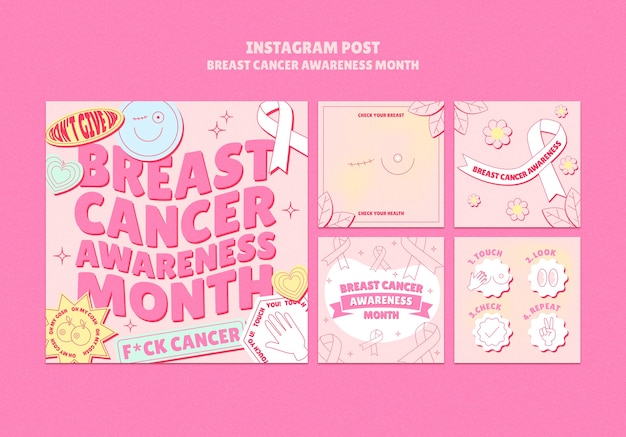Here is a cleaned-up and detailed caption for the described image:

---

This promotional image is designed to raise awareness for Breast Cancer Awareness Month. It features a bright pink background, drawing immediate attention. At the top, in tan-colored text, the headline reads "Instagram Post: Breast Cancer Awareness Month."

Below the headline, there are five smaller images. The largest image, positioned on the far left, features a yellow oval with bold red text that encourages with the words "Don't Give Up." In the center of this image, pink text reiterates the theme: "Breast Cancer Awareness Month." At the bottom, a striking white banner displays the phrase "Fuck Cancer," emphasizing the fight against the disease. Additionally, there is a pattern in the bottom-left corner with repeated "Oh my gosh" text in red within a yellow star icon, adding a layer of emphasis.

Toward the right of this main image, various smaller images provide different messages and illustrations:
- One image boldly states "Breast Cancer Awareness Month."
- Another image, incorporating a white ribbon, reads "Breast Cancer Awareness."
- A graphic advises, "Check Your Breast, Check Your Health," depicting a breast with a noticeable absence of one, symbolizing the impact of breast cancer.
- In the bottom right corner, an image outlines a self-check routine with steps: "Touch, Look, Check, Repeat."

Decorative elements such as a little heart at the top and a smiley face add a touch of positivity and hope throughout the composition. Overall, this vivid and comprehensive collage is geared towards spreading awareness and encouraging proactive health measures during Breast Cancer Awareness Month.

---